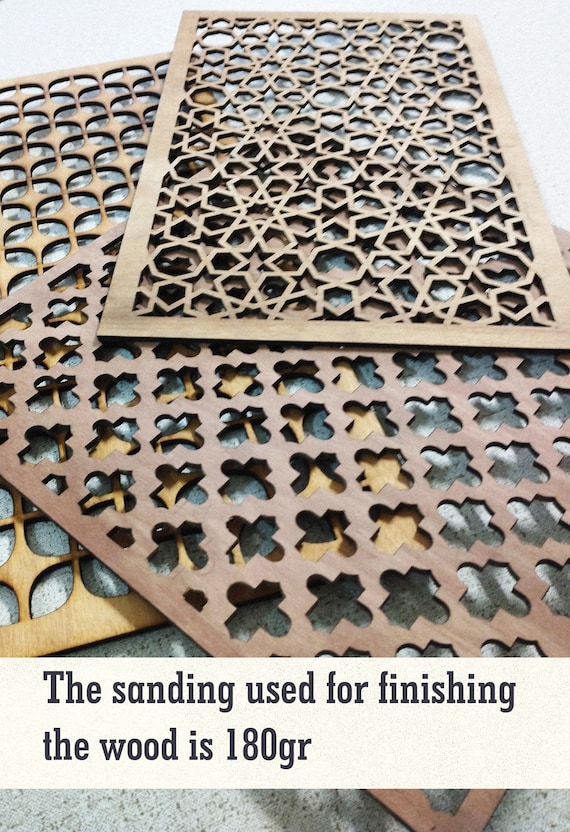This vertically oriented photograph showcases an arrangement of three thin, rectangular wooden panels lying on a beige, splotched surface. These panels, each approximately half an inch thick, 12 inches wide, and 2 feet tall, are adorned with intricate, geometric designs. The wood displays varying shades of medium to light brown, emphasizing the natural diversity of the material. The patterns carved into these panels include stars, hexagons, swirling motifs, irregular circular shapes, diamonds, and crosses, with each panel featuring unique and symmetrical designs. A beige text box at the bottom of the image indicates that the sanding used for finishing the wood is 180GR, providing a technical detail that enhances the appreciation of the craftsmanship.